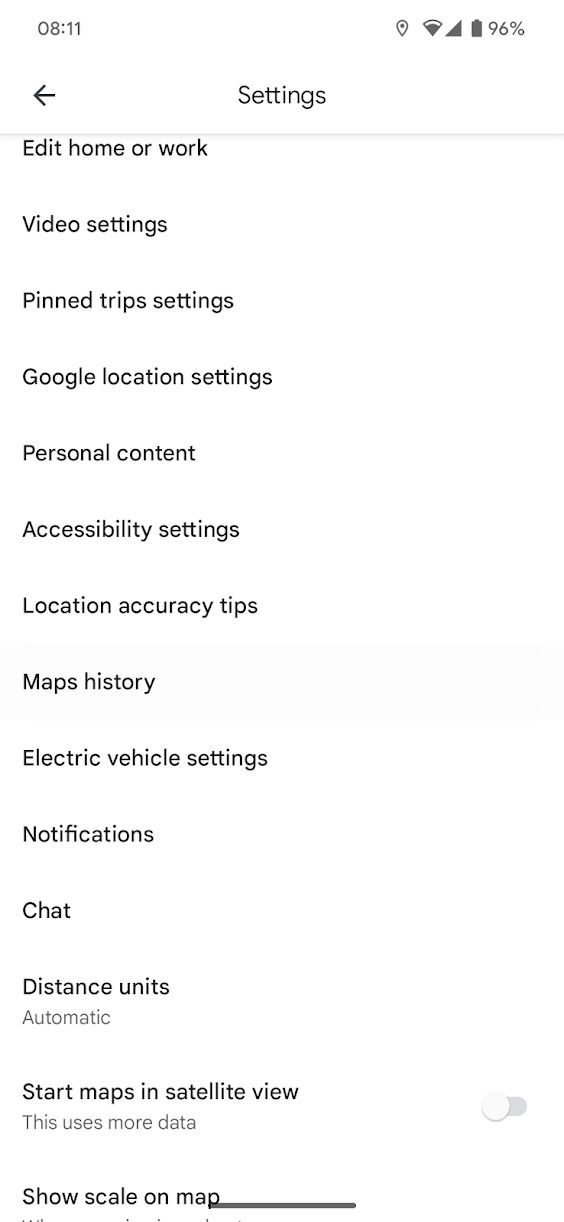The screenshot depicts the settings screen of a mobile device. The current time displayed in the upper left-hand corner is 8:11 AM. To the right, a series of icons provide additional status information: the battery at 96%, Wi-Fi signal strength, cellular signal strength, and location services active. 

The screen features a light gray background, with the primary text in black. The screen title reads "Settings," indicating the various customization options available. 

The settings options listed are:

- Edit Home or Work
- Video Settings
- Pin Trip Settings
- Google Location Settings
- Personal Content
- Accessibility Settings
- Location Accuracy Tips
- Maps History
- Electric Vehicle Settings
- Notifications
- Chat
- Distance Units (currently set to "Automatic" in gray subtext)

Further options include toggles for "Start Maps in Satellite View," which is currently off with a note in gray text stating "This uses more data," and "Show Scale on Map," presented in black text. This comprehensive list provides users with various ways to personalize their mobile experience.